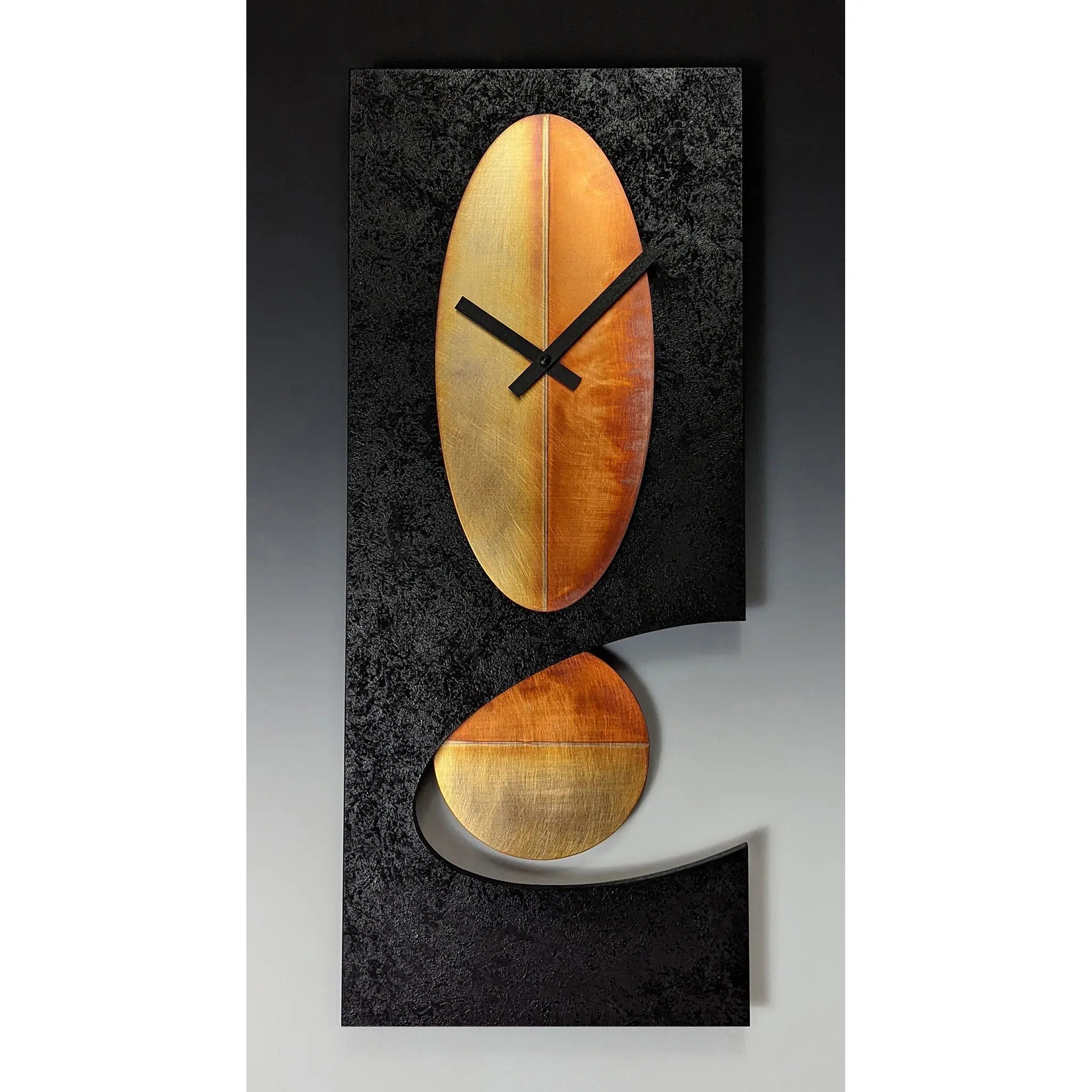This photograph features an abstract, vertically-oriented art piece designed to resemble a modern clock mounted on a gray wall. The main body is made of textured black metal, which appears taller than it is wide. The black surface has intricate designs and a semi-elliptical cut-out near the bottom, through which a copper-colored, round pendulum is visible. This pendulum contrasts with the darker tones of the metal frame. The upper part of the clock features an oblong, egg-shaped clock face, also copper in color with a gradient that lightens towards its center and darkens along the seams and edges. This face lacks numbers and features two thin, black hands indicating the time at approximately 10:10. The overall composition, including the cut-out shapes and the metallic textures, reinforces the abstract aesthetic of this unique timepiece.